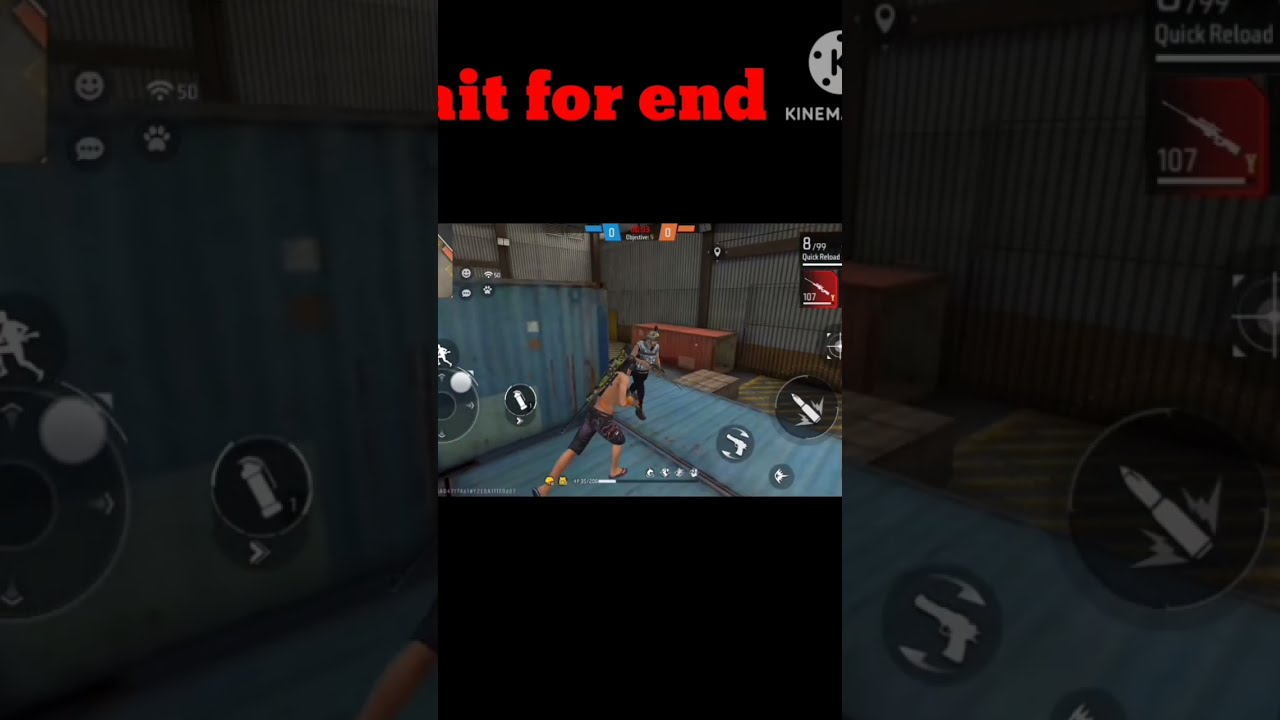The image is a wide rectangular screenshot of a mobile video game displayed in a portrait format. It is split into three vertical sections: the left and right sections are darker, zoomed-in close-ups of the center section, which is the main gameplay area. The center section is bordered by thick black bars at the top and bottom. At the top, partially cut-off bold red text reads "ITFOREND" and in gray capitals to the right, it says "KINEM." The gameplay shows a character wearing jean shorts, flip-flops, and a skimpy shirt standing on blue and gray storage containers inside a warehouse. The character has a gun on their back and is holding another gun. Another armed character wearing a white shirt or vest is approaching. The screen features mobile game controls including a left-side analog stick and right-side action buttons with icons of a gun and a bullet. The entire setup suggests it could be a multiplayer game.